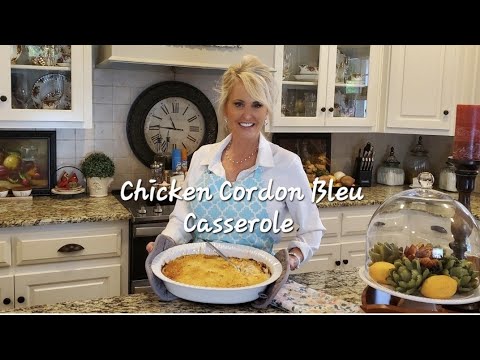In this detailed video still from either a TV program or a YouTube video, a Caucasian woman in her 40s with blonde hair stands smiling in a well-appointed kitchen. She wears a diamond-pattern blue apron over a white blouse and has a necklace around her neck. Her hair is pinned up neatly. The woman is holding a white casserole dish, labeled with text that reads "Chicken Cordon Bleu Casserole." She wears oven mitts, suggesting the dish has just been taken out of the oven.

The bright, inviting kitchen features white cabinets, some with glass fronts revealing ornamental chinaware. An island counter with a fruit casing and marble countertops are also visible, along with various pots, pans, seasoning containers, sugar containers, and knives neatly arranged on the countertops. A large clock is prominently displayed on the wall above the stove, and a candle in a candle holder adds a homely touch. To the right of the woman, there is a glass dome containing succulents, contributing to the kitchen’s decorative elements. The overall scene is warm and inviting, framed by the woman's joyful expression as she presents the freshly prepared chicken cordon bleu casserole.